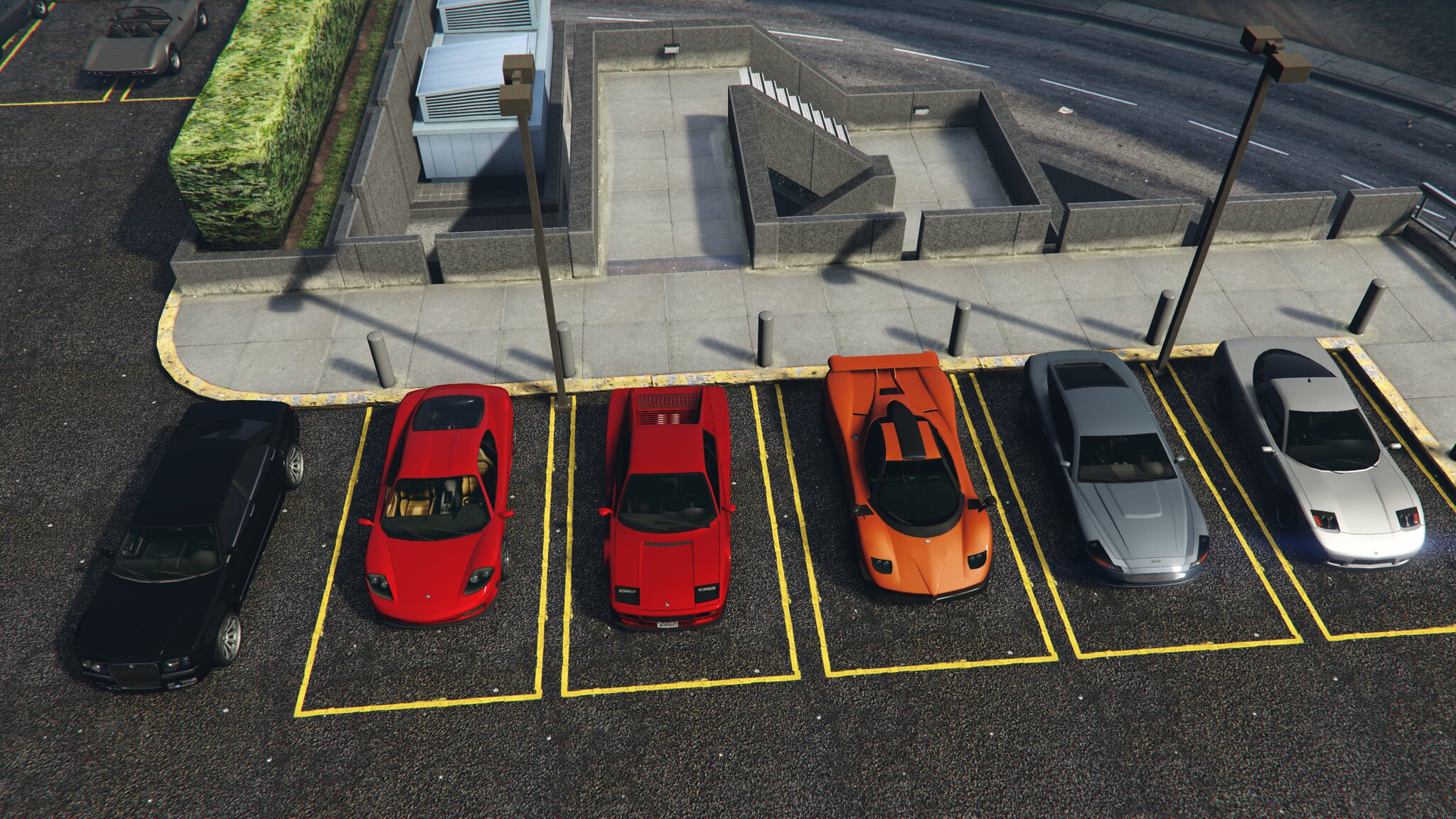This image is a detailed, horizontally oriented color snapshot taken from above, depicting a highly realistic model parking area, possibly from a video game such as Grand Theft Auto V. The parking lot is asphalt with speckles of white dots and features a row of six luxury supercars meticulously parked and arranged. 

From left to right, the cars include a glossy black car, two vibrant red sports cars, an opulent orange car, and two sleek gray cars. Five of these cars are neatly situated within yellow-bordered parking spaces, while the black car on the far left is slightly outside of a designated space. 

The parking area is bordered by a sidewalk made of concrete, accompanied by a gray stone pathway and staircase that leads down to a highway with white dashed lines. Additionally, there is a hedge row running parallel to the parked cars, enhancing the layout's realism. The entire scene is surrounded by what appears to be a racetrack, reinforcing the high-end, supercar theme of the setting.